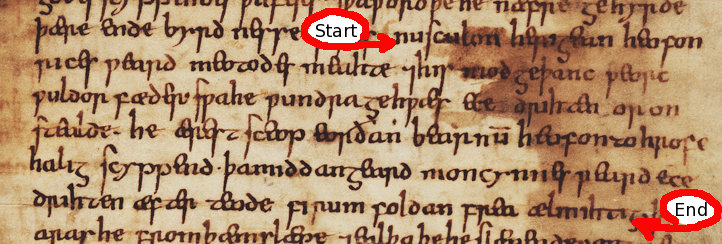The image showcases a highly aged and worn fragment of a manuscript, possibly originating from the medieval period, indicated by its historical script and archaic language, likely English or Latin. The manuscript page, now beige and discolored with time, exhibits characteristics of old-fashioned writing styles. Notably, the image contains digital annotations in the form of two red, oblong-shaped arrows filled with white, labeled "start" and "end," demarcating specific points within the text. Given the symbols and letters, there is a suggestion that the manuscript might mimic the alphabet from the Lord of the Rings universe, hinting at it potentially being a movie prop. The "start" arrow appears in the upper middle section, while the "end" arrow is positioned towards the lower right corner of the image.